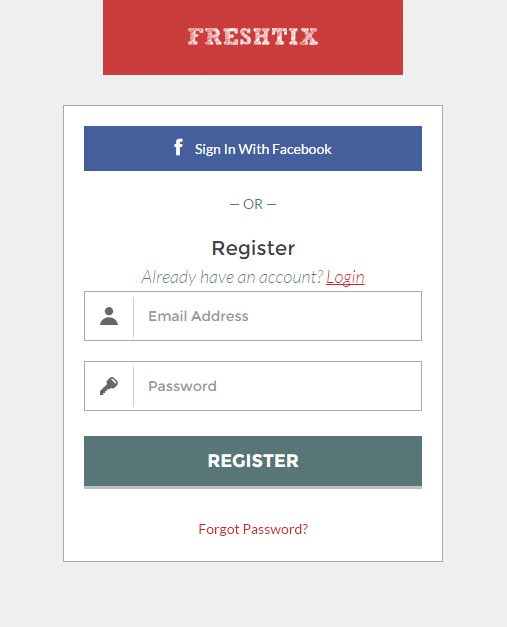This image captures the screen of a cell phone displaying a registration and login interface for an application named **"Freshtix."** At the top, a red box prominently displays the app's name: **"Freshtix"** in white text.

Below, there is a white rectangular area containing different login and registration options. At the top of this rectangle, there is a blue button with a white **"F"** symbol, representing Facebook, and text that reads: **"Sign in with Facebook."** 

Underneath this option, there is a horizontal dash followed by the word **"OR"** in capital letters, flanked by two more dashes. 

Below that, in black print, is the option to **"Register."** Directly beneath this, it says **"Already have an account?"** followed by **"Log in"** in red, underlined text, indicating that it's a clickable link.

Moving further down, a grey rectangular box contains a silhouette of a person and the text **"Email address."** Beneath this, another rectangle shows a key icon followed by the word **"Password."**

At the bottom of this area, a green rectangular button with white text reads **"Register."**

Finally, at the very bottom of the screen, in red print, the text **"Forgot password?"** is displayed, indicating another clickable option.